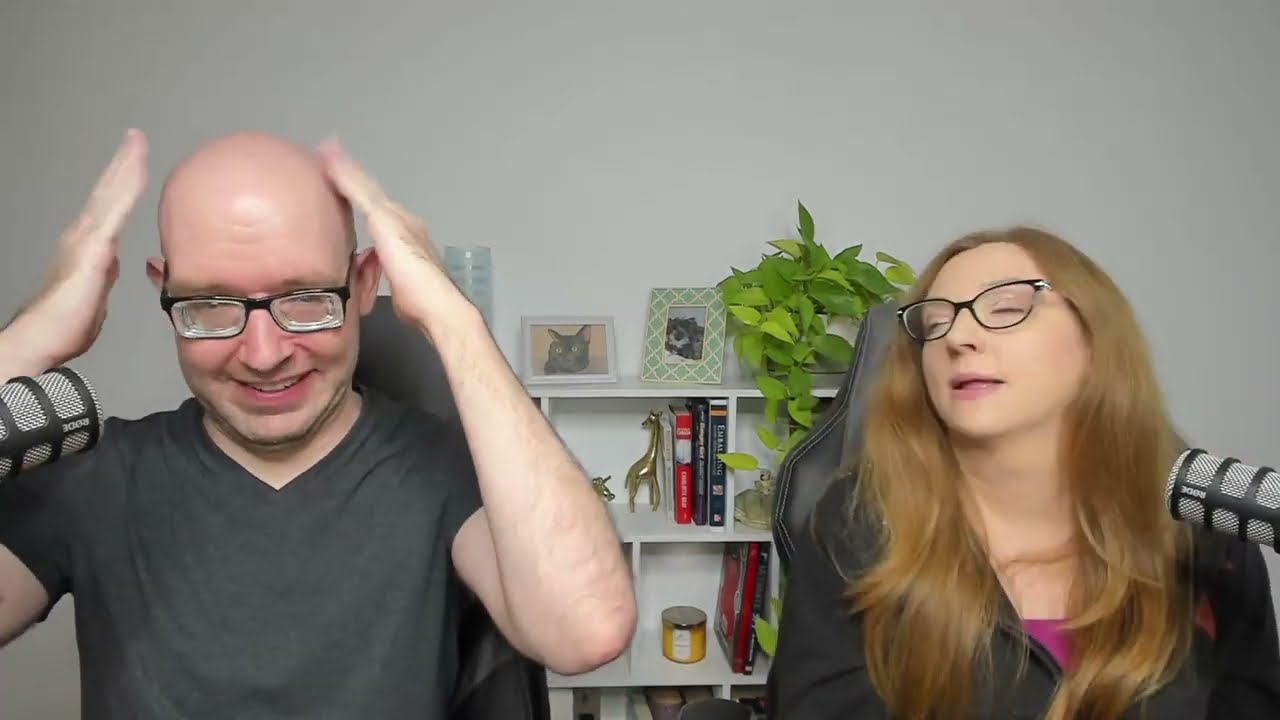This is a horizontal color photograph capturing an indoor setting featuring two people, both engaged in a podcast. The style is photographic realism. On the left side of the image is an adult white man, bald-headed with black-rimmed, thick-lensed glasses. He is wearing a gray v-neck t-shirt and has his hands near his head while smiling broadly. To his right, a silver and black microphone is visible. 

On the right side of the image, there is a white woman in her thirties or early forties with long, wavy blondish-brown hair. She is wearing black-rimmed glasses, a black jacket, and a purple sweater. Her eyes are closed, and her mouth is open, possibly mid-speech, with a slight smile. A similar microphone is positioned to her left.

The background features a white or light gray wall against which a white bookshelf stands. The bookshelf contains three shelves adorned with various items including books, a giraffe bookend, and a yellow candle. The top shelf has a green plant and two framed photographs of cats. The mid-tier shelf underneath the giraffe bookend holds additional unidentifiable books and what appears to be a candle.